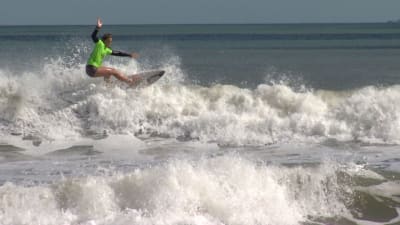In the image, a surfer is skillfully riding a grey and white surfboard amidst small crashing waves. The surfer, who appears to be Caucasian, is dressed in a vibrant teal neon green shirt with black sleeves and gray shorts. With their arms raised to maintain balance, they navigate through the frothy white waves that are splashing in all directions. The background of the photograph showcases the ocean's distinctive greenish-blue hue and a grayish sky above, adding a dramatic tone. Closer to the bottom of the image, calmer stretches of water can be observed with bubbles visible in the tinted water on the right side, highlighting the dynamic interplay between the still and turbulent sections of the sea.